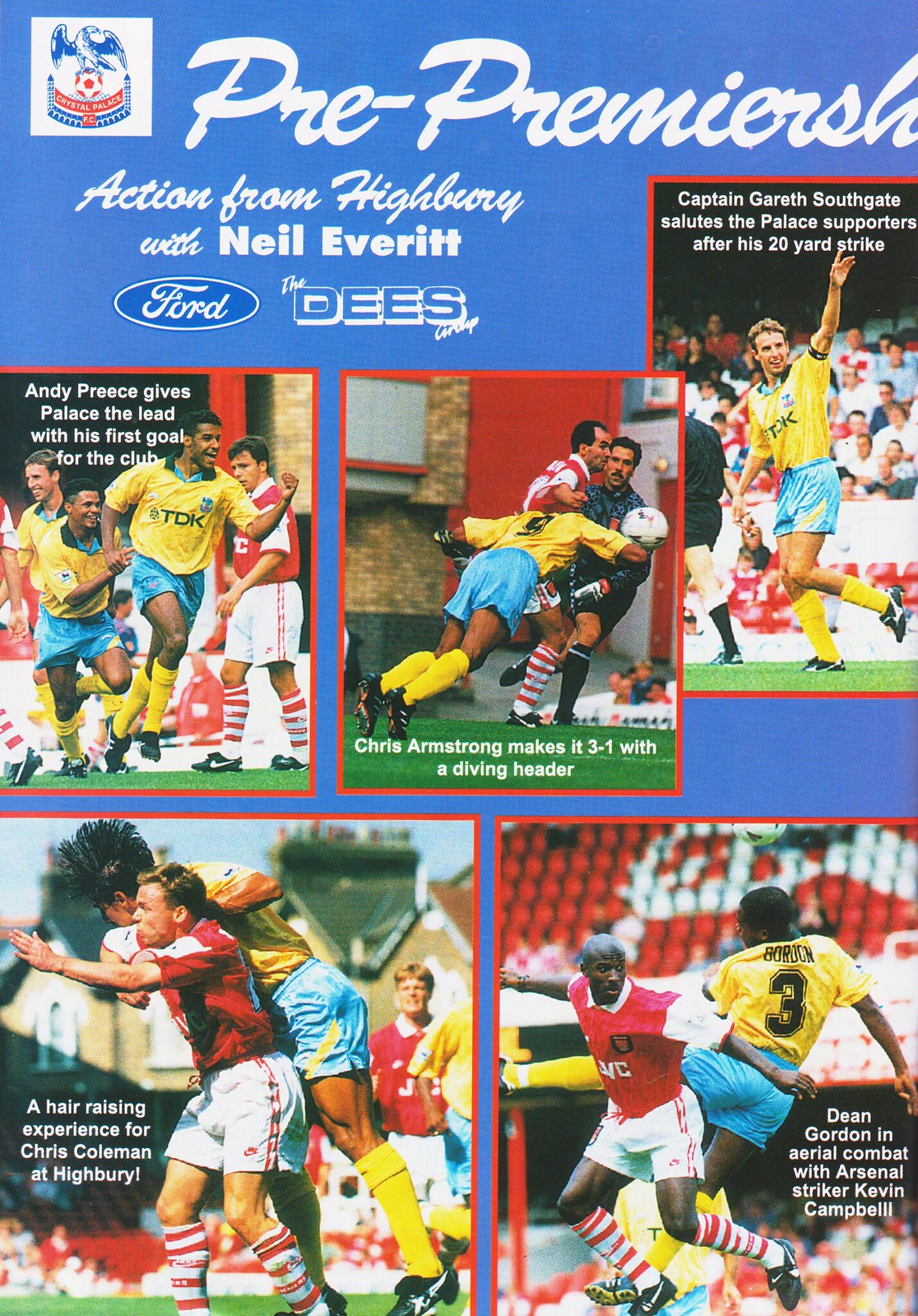This vintage soccer pamphlet or advertisement, designed in a collage format, prominently features five images capturing dynamic moments from a soccer match at Highbury. The top banner displays the phrase "Pre-Premieres Action from Highbury," accompanied by the iconic blue and white Ford company logo and the name Neil Everett.

In the first image on the top left, the caption reads, "Andy Priest gives Palace the lead with his first goal for the club," featuring players in yellow and blue uniforms facing off against those in red and white. The second image features Chris Armstrong in action, with the text, "Chris Armstrong makes it 3-1 with a diving header," against a backdrop of brown and tan brick buildings.

The third image spotlights Captain Gareth Southgate, with the caption, "Captain Gareth Southgate salutes the Palace supporters after his 20-yard strike," celebrating in the same yellow and blue kit. 

Below these, the leftmost bottom image highlights, "A hair-raising experience for Chris Coleman at Highbury," showcasing the intense play. The final image to the right captions, "Dean Gordon in aerial combat with Arsenal striker Kevin Campbell," both players caught in mid-air during a challenging play.

The pamphlet is a vivid depiction of soccer excitement, capturing key moments and players, with detailed text on each image to enhance the viewing experience.